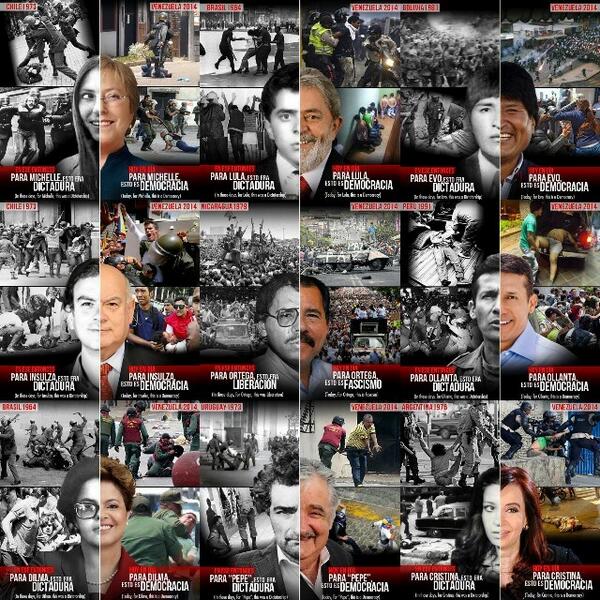The image is a poignant collage depicting police brutality across various countries, including Chile, Venezuela, Brazil, Peru, and Argentina, with additional nations labeled in red but blurred. The collage features numerous distressing photographs of individuals being assaulted or forcibly subdued by police officers. These officers are often dressed in navy uniforms, highlighting the widespread nature of such violence.

Prominent political leaders from these countries are also displayed in the forefront of the image, though only partially visible. Each photograph within the collage captures the visceral reality of police misconduct, with specific scenes showing individuals being beaten or dragged by force.

The upper left corner of the collage shows a person on the ground being beaten by police, while the bottom right corner depicts another person being forcibly dragged. In total, nine leaders are identifiable within the image, juxtaposed against the backdrop of brutality to emphasize the tension and suffering under their regimes. The collage powerfully communicates the grave issue of police violence and the human impact of political repression.